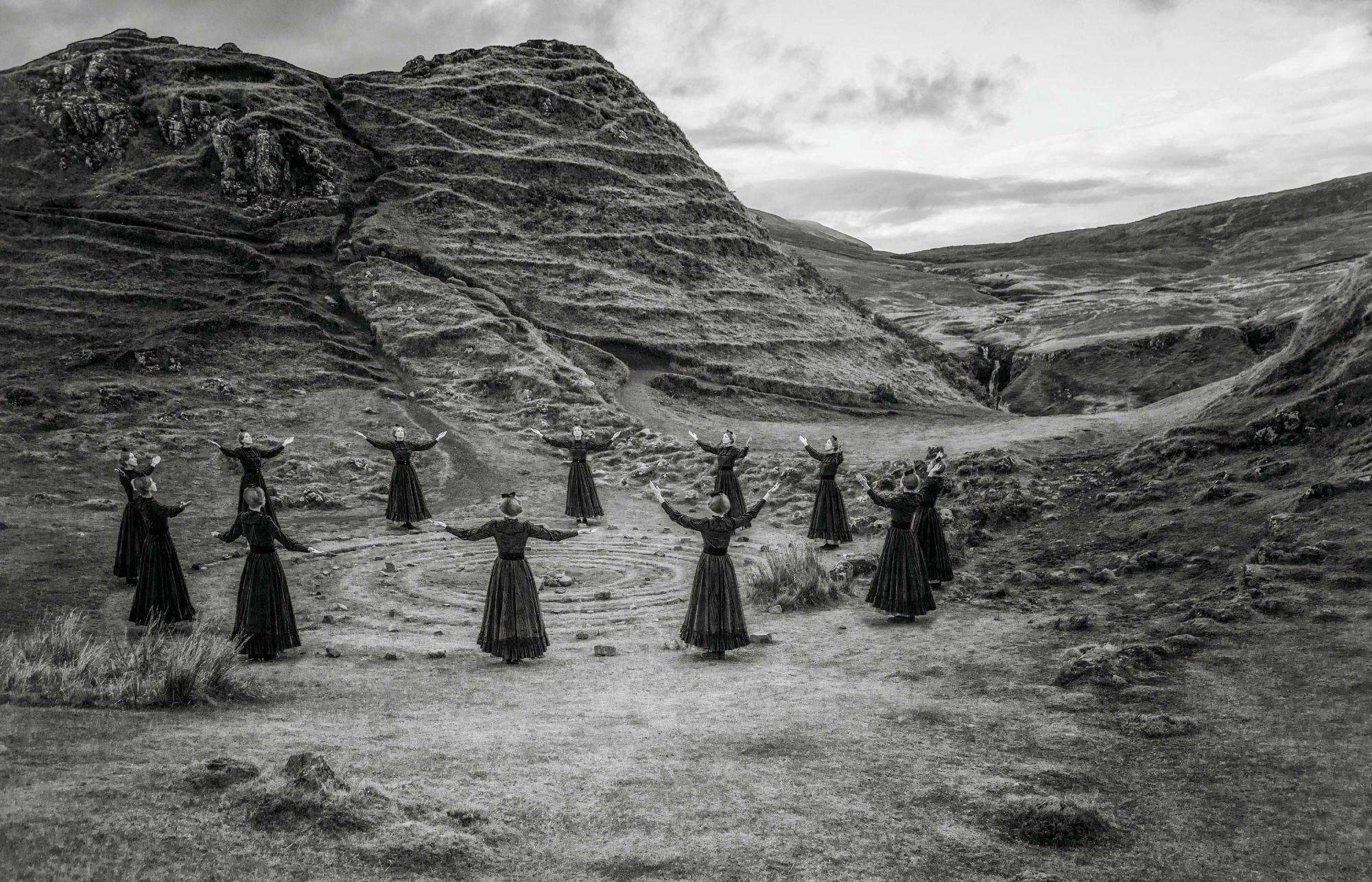In this black-and-white photograph, a group of 12 women stands in a wide circle in a stark, rugged landscape, possibly dominated by rock and lacking much plant life. Each woman is wearing a matching ankle-length, long-sleeved black dress and has her hair styled into a bun, topped with some unclear head accessory. Their arms are outstretched upwards, with palms facing the sky, as if in a prayer or ritualistic gesture. Concentric rings appear on the ground within their circle, leading to a central point with an indistinct object. The background reveals a sizable hill or small mountain, contributing to the sense of isolation in this natural setting. Enhanced by a slight vignette effect, the sky appears light with scattered clouds, adding a somber, timeless quality to the scene.